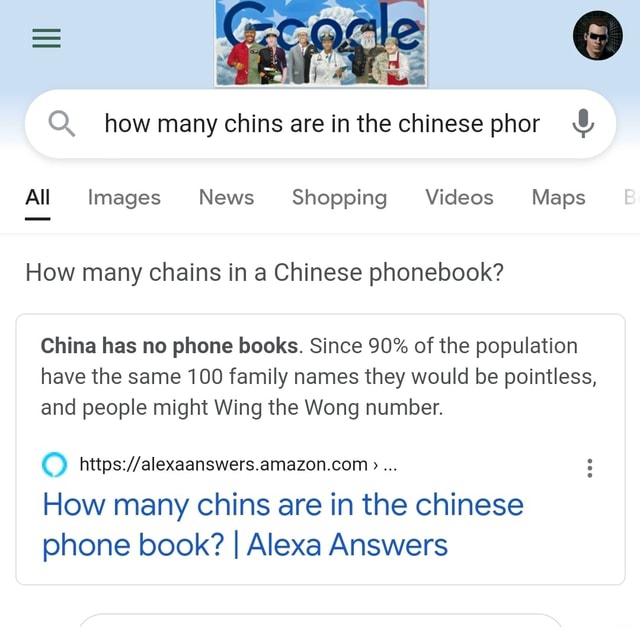This image appears to be a screenshot of Google search results with a distinctive Google Doodle commemorating either Veterans Day or Memorial Day. The background, a pale blue gradient fading to white, features an illustrative Google logo adorned with patriotic American motifs, including stars, stripes, and clouds. Saluting this design are six uniformed members of various U.S. military branches, portrayed both as veterans and active personnel, showcasing diversity in terms of age and ethnicity.

In the top right corner, a user’s avatar is displayed—a circular image of a Caucasian man with short black hair and dark sunglasses. Centered below the logo is a Google search bar outlined in white. To the left of this bar is a magnifying glass icon, and within the bar, the search query is displayed in black text: “how many chins are in the Chinese PHOR,” accompanied by a microphone icon on the right.

Directly beneath the search bar are clickable options in gray text, starting with an underlined "All" in black, followed by "Images," "News," "Shopping," "Videos," and "Maps." The beginning of a partially visible option starting with the letter "B" suggests additional categories are available off-screen.

Following these options is a thin gray bar, below which the query “how many chins in a Chinese phone book” appears in bold black letters. Encased in a faint gray box, the response reads: "China has no phone book, since 90% of the population have the same 100 family names it would be pointless, and people might be winged with the wrong number." The source of this information is identified as https://alexaanswers.amazon.com, adjacent to a sideways pointing "V" and an ellipsis arranged vertically.

A bold hyperlink in blue text highlights the phrase "how many chins are in the Chinese phone book," followed by the logo for Alexa Answers within a blue bar. At the bottom of the image, an upper portion of another search result is partly visible as a gray oval, cut off by the edge of the screen.

Overall, the screenshot captures a Google search result page with a topical Doodle likely related to a U.S. patriotic holiday, highlighting a peculiar query and its resulting answer from Alexa Answers.